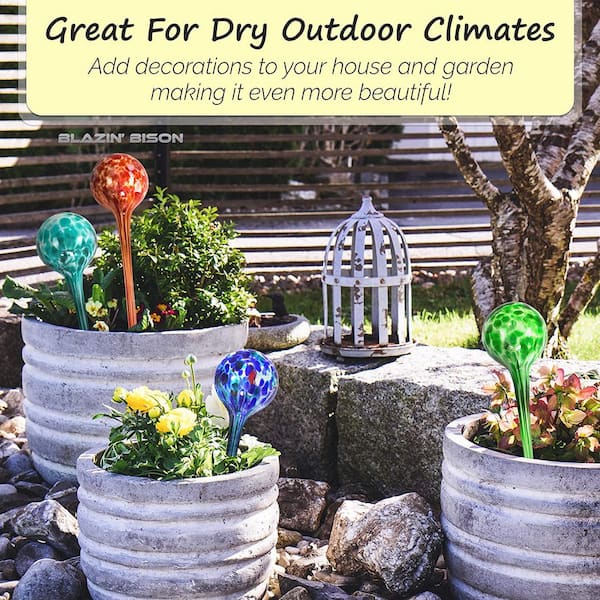This photograph captures a charming garden area, possibly someone's backyard, designed for both functionality and aesthetics. At the bottom, there is a stone-covered section featuring several grey or brown stones. Atop these stones are three large, grey-colored, concrete flower pots. Each pot hosts various plants, some of which are adorned with yellow flowers amidst green leaves. Among the plants, there are colorful, round decorative items with sticks at their bases, available in green, blue, and red tones. Additionally, large glass bulbs designed to maintain consistent watering are inserted into the soil in each pot. A small stone wall, made up of two substantial rectangular stones, provides a quaint structure, which also holds a distressed, antique-looking birdcage for decorative purposes. Extending from this section is a lush green grass area featuring the trunk of a tree. In the background, a wooden fence completes the cozy garden ambiance. The top part of the image displays a horizontal banner. While there's some discrepancy in the text color—green or yellow—the message is clear, reading: "Great for dry outdoor climates, add decorations to your house and garden making it even more beautiful."